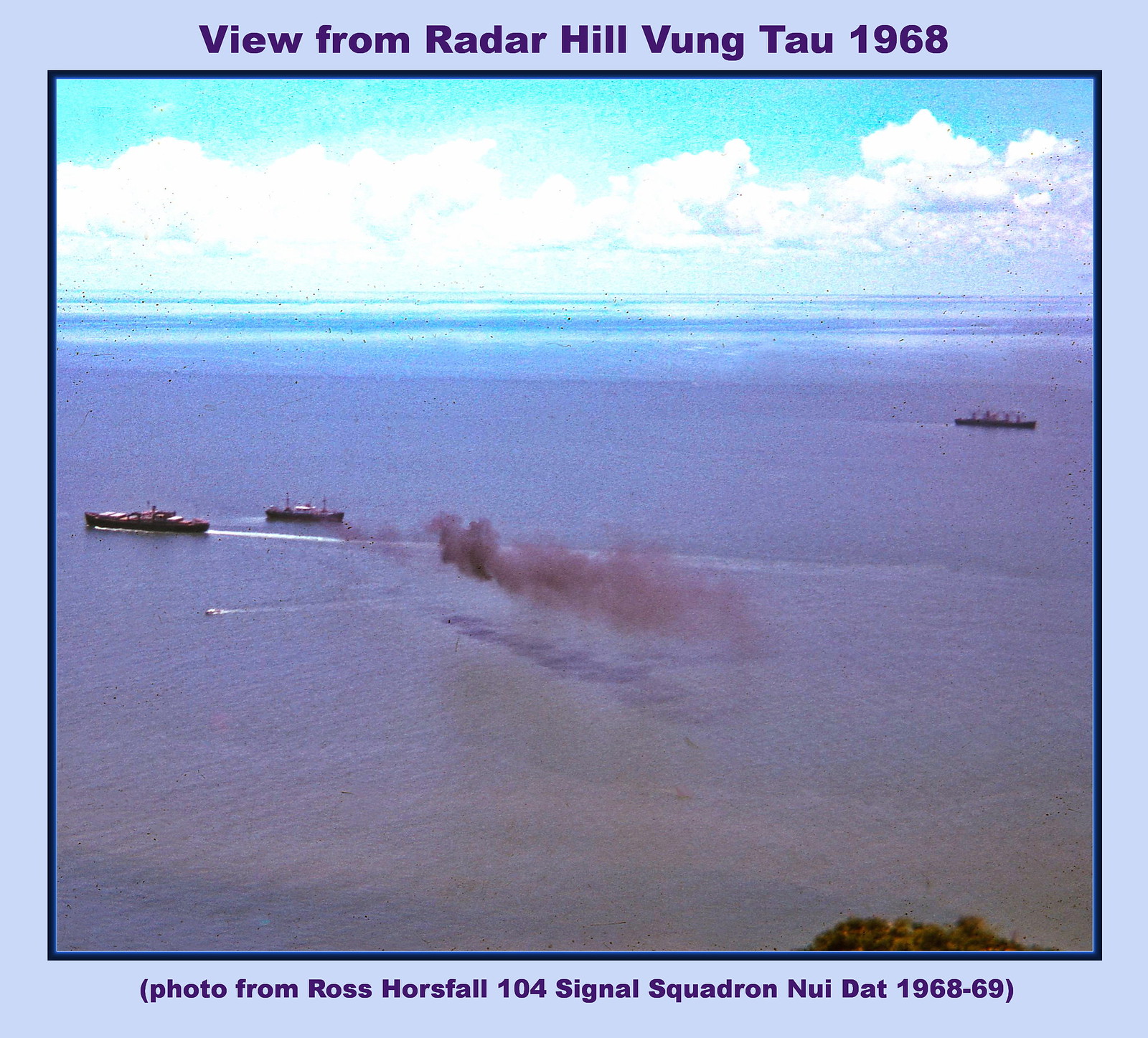Here's the detailed caption, combining and cleaning up the descriptions:

This image resembles a vintage postcard and features a photograph taken in 1968 at Radar Hill, Vung Tau, Vietnam. The image is framed by a light purple outline, with text at the top in dark purple lettering reading, "View from Radar Hill, Vung Tau, 1968." Below, a detailed scene of the coastal area is depicted. The photograph shows a vast body of water, likely leading out to the ocean, under a partly cloudy sky. Three ships are visible on the water: one in the distance on the left side, and two others heading out of the frame on the right, with a plume of smoke trailing from one. The horizon is dotted with clouds, and the bottom right corner of the image displays some vegetation, hinting at the shoreline. Additional text at the bottom, in matching dark purple font, reads, "Photo from Ross Horsefall, 104 Signal Squadron, Nui Dat, 1968-69." The image appears damaged and oversaturated, contributing to its vintage aura.